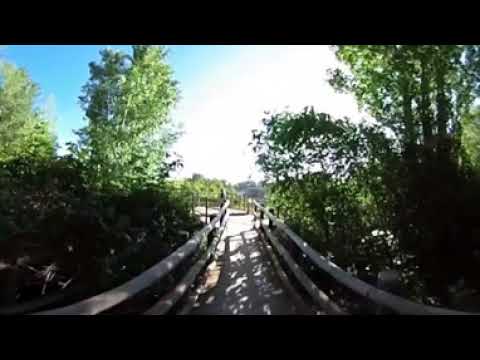The photograph depicts a natural setting, likely from a park or a forest trail, featuring a light brown wooden footbridge with cylindrical log railings on both sides. The bridge starts at the bottom center of the image and runs vertically, leading to the middle of the picture where it seemingly ends, possibly at an overlook. The bridge surface is made of wooden planks, possibly worn and in need of replacement over time. Dense trees flank the bridge on both sides, casting ample shadows across its path, creating a serene and shaded ambiance. The backdrop above the canopy of trees reveals a partly cloudy sky with patches of light blue. Although the image is blurred, hinting at an air of mystery, there is no clear indication of the bridge’s termination point, whether it be another set of trees or some unseen structure.